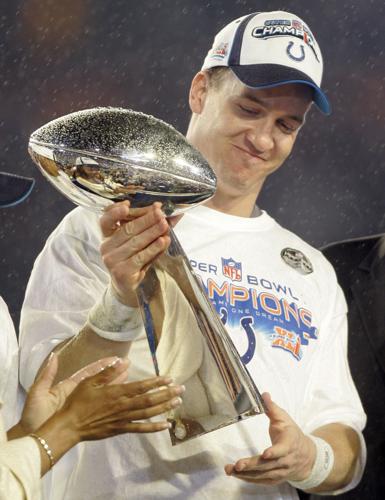In this detailed outdoor photograph, Peyton Manning proudly holds the gold and reflective silver Super Bowl trophy, its iconic football shape glistening with raindrops under a dark gray, blurred backdrop suggesting it’s raining. Manning stands at the center, wearing a white T-shirt and a white hat, both emblazoned with “Super Bowl Champions” and featuring the blue horseshoe logo of the Indianapolis Colts. He appears joyful, perhaps aged 25 to 30, celebrating the victory. In the bottom left corner, a pair of clapping hands, likely belonging to a black woman wearing a bracelet, further evokes the celebratory atmosphere of this triumphant moment.